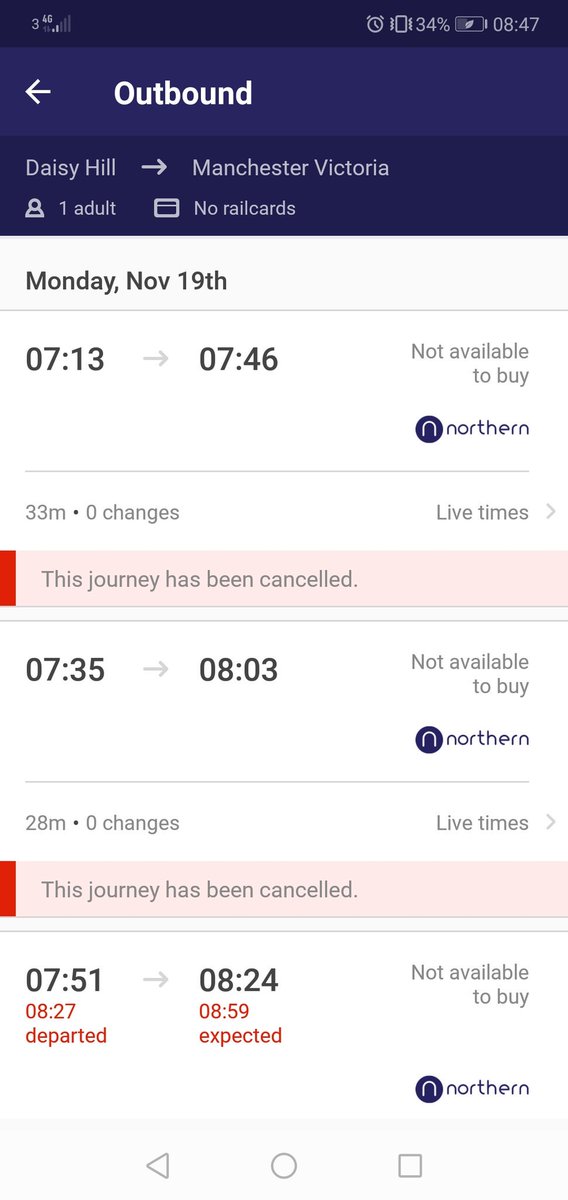Screenshot of a travel app interface displaying several train journey options and statuses:

- At the top, there is a status bar showing a vibration icon, 34% battery, and the time (8:47) with a clock icon.
- Below this, a blue banner with a lighter blue streak that displays "Outbound" and a back button.
- The screen shows a route from Daisy Hill to Manchester Victoria with a right arrow in between.
- An icon indicates one adult traveler, and the text mentions no railcards being used.
- There’s a credit card icon beneath this information.
- The date is Monday, 19th of November, displayed against a white background, indicating the journey is from 7:13 AM to 7:46 AM, a total duration of 33 minutes, with zero changes. However, it notes that the ticket is not available for purchase on Northern Rail.
- A red bar with a pink stripe across announces that "this journey has been cancelled."
- Below, another schedule indicates a journey from 7:35 AM to 8:03 AM, for 28 minutes with zero changes, also not available to buy on Northern Rail and marked as cancelled.
- The third listed option shows a journey from 7:51 AM to 8:24 AM. It departed at 8:27 AM and is expected to arrive at 8:59 AM. Again, this journey is not available to buy on Northern Rail, with red text indicating the departure and arrival times.
- At the bottom of the app, there are back and close buttons. 

The overall app design is described as clean, simple, and effective.